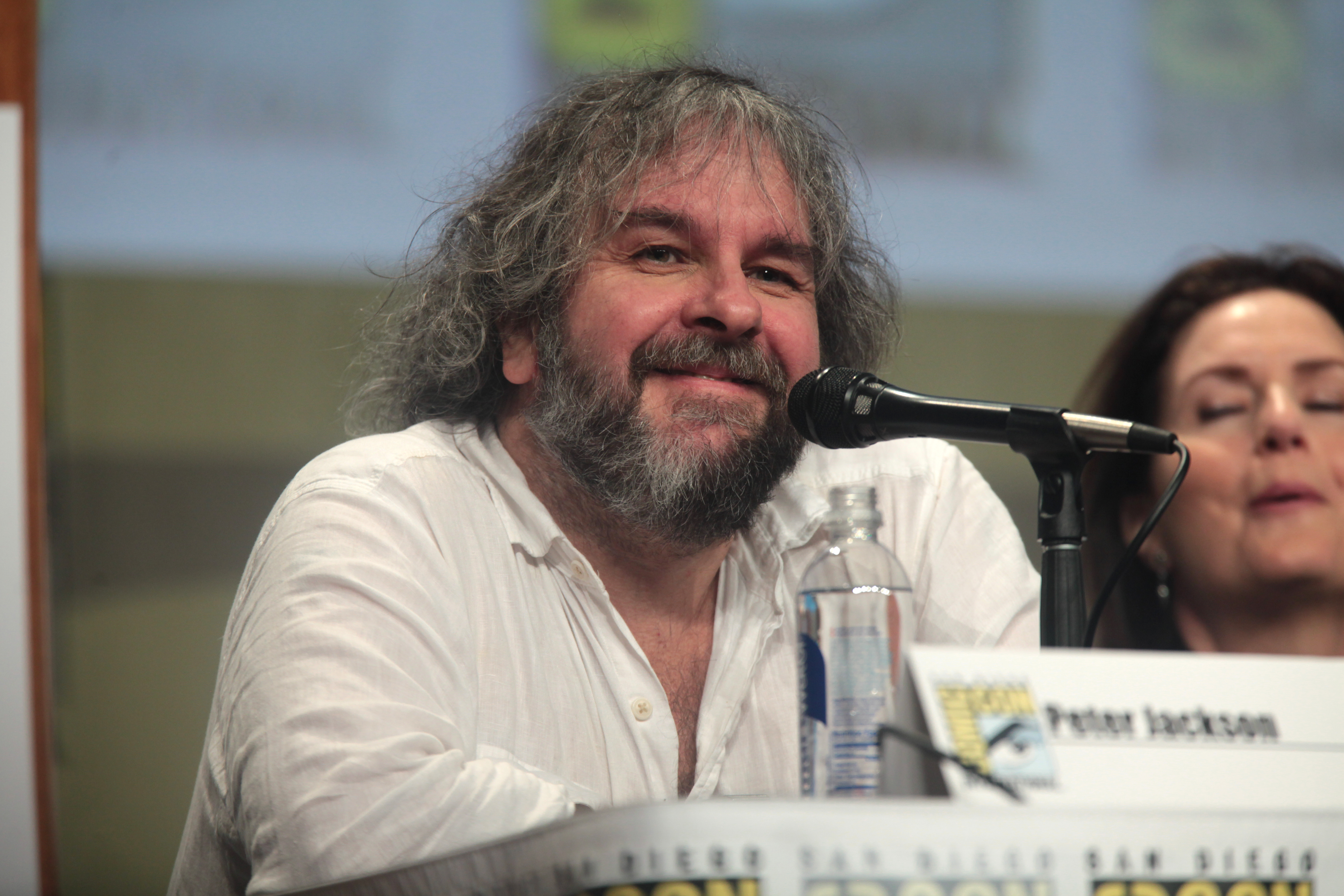In the image, Peter Jackson is seated at a table in front of a microphone, possibly at San Diego Comic-Con. He has long, frizzy gray hair that falls to his shoulders, paired with a bushy, predominantly gray beard speckled with darker shades. He wears a white button-down shirt with the top buttons undone, revealing some chest hair. A name card reading "Peter Jackson" is placed in front of him. On the table before him, there is a clear plastic water bottle, which resembles a Smartwater bottle without its cap. To his right, a woman with dark brown hair and partially closed eyes sits with her mouth slightly open. The blurry background features a mostly whitish color with hints of yellow and a darker brown stripe at the bottom, possibly part of the San Diego Comic-Con logo.